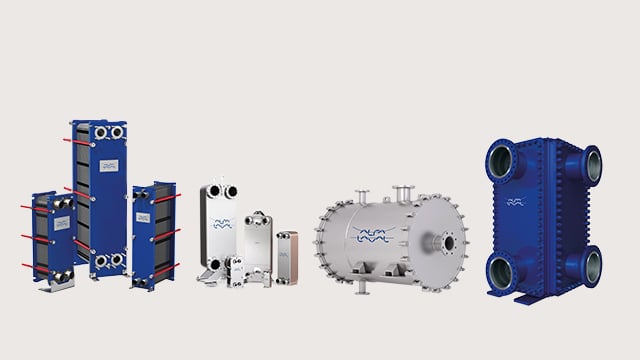This color photograph showcases an array of small machinery components arranged from left to right. Starting on the left, there are three blue, square-like pieces, resembling upside-down drawers or toolboxes, each interconnected by slender red rods and featuring round black grommets. Adjacent to these are three shiny metallic pieces, which also include circular grommets arranged in pairs at the top and bottom. Further to the right is a cylindrical object made of gleaming silver metal, adorned with rivets along its edges. Finally, on the far right, stands a blue rectangular 3D object, punctuated by large circular holes, reminiscent of the grommets seen earlier, potentially designed for cable connections or component fittings. Each piece exhibits intricate design details, emphasizing their utilitarian yet complex nature.